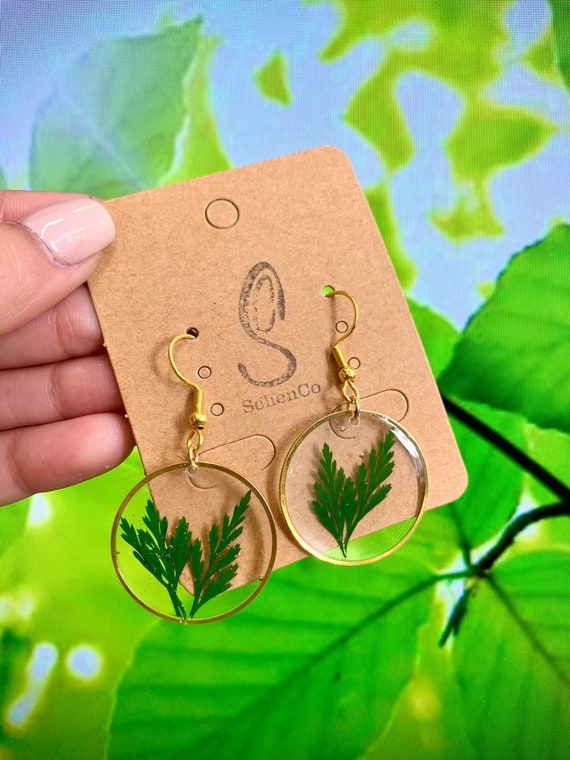The photograph, oriented in portrait style, prominently features a close-up of a left hand wearing pink fingernail polish on the thumb. This thumb, along with the fingers, holds a kraft brown marketing placard at a slight angle to the left. The placard, stamped with an elegant letter "S" and the brand name "Solean Company" beneath in subtle script, displays a pair of handcrafted, dangly earrings. These earrings, attached by gold French hooks to the placard, boast large circular frames of gold. Encased within each frame is clear resin embedding two vibrant, dark green leaves, resembling delicate ferns. The resin gives a magnified view of the leaves, which stretch out within the confines of the gold circle, touching the inner edges. The background of the image is slightly blurry, featuring an outdoor-like scene with a vivid blue sky and lush green leaves, enhancing the artisanal quality of the earrings.